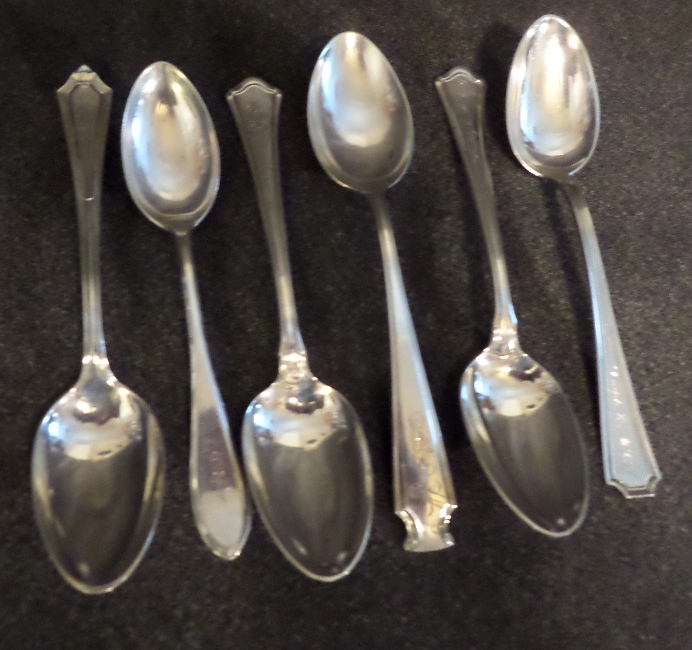The image portrays six antique-style silver spoons arranged on a dark gray background, possibly a speckled countertop or table surface. The spoons alternate in position: starting with the first spoon facing downward, the next upward, in a rotational pattern. They differ in size, alternating between large and small, with three of each. Each spoon exhibits unique, ornate designs on their handles, which range from pointed to rounded tips and feature intricate patterns and possible inscriptions. The large spoons appear to have water droplets on them, adding a touch of realism to the slightly blurry picture. This detailed arrangement and the vintage aesthetic of the spoons suggest they belong to different collections, lending a nostalgic, antique quality to the scene.